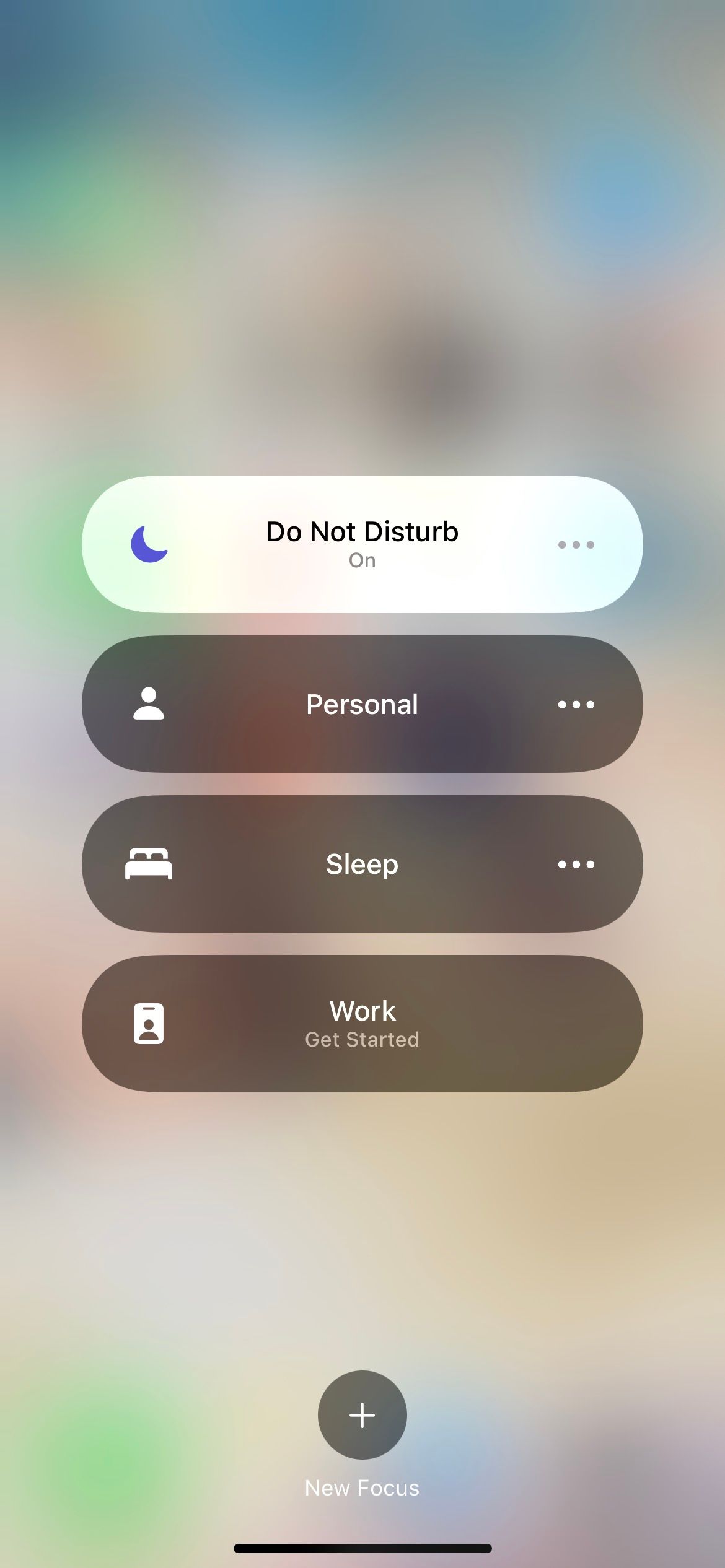The image displays four selectable options prominently centered against a blurred background with hues of green, brown, and blue. The background also features a transparent black overlay for a focused visual hierarchy. 

1. The topmost option, "Do Not Disturb," is highlighted with a slightly white background and black text. It has a blue half-moon icon to its left and a horizontal three-dot menu icon on the right, indicating it is currently active.
 
2. The second option, "Personal," displays a white profile icon on the left and a similar three-dot menu icon on the right. The text is white, indicating it is not selected.

3. The third option, "Sleep," features a white bed icon on the left side, and the standard three-dot menu icon on the right, also in white, indicating it is unselected.

4. The fourth option, "Work," prompts the action "Get Started" and includes a white work tag icon on the left, with the white three-dot menu icon on the right.

At the bottom of the center area, there is a circular button with a plus sign inside, labeled "New Forecast." All unselected options and icons are rendered in white except for the selected option's blue half-moon icon.